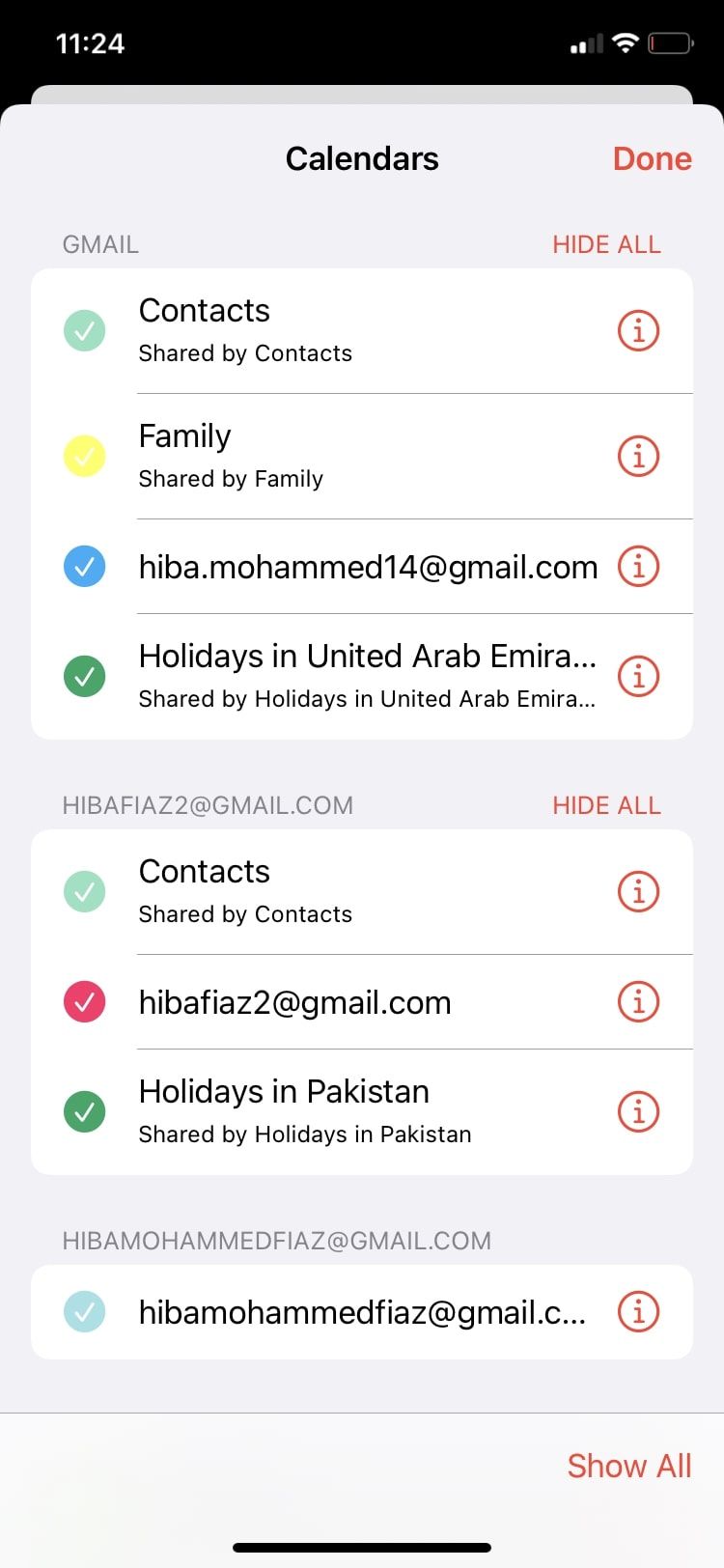This image is a detailed screenshot from an iPhone's mobile device screen. At the top of the display, the status bar reveals critical information: the battery indicator is in the red zone with a single bar remaining, signaling that the phone is about to run out of battery. The device shows a full Wi-Fi signal and two bars of cellular reception. The time displayed is either 11:24 a.m. or p.m. (the exact time of day is not specified).

The screenshot captures the settings interface, specifically the general settings section within the calendar settings. Dominating the screen is a white pop-up window labeled "Calendars" at the top. A red "Done" option is available next to this label, presumably to exit the settings after making changes.

Below the header, the screen is divided into sections by different accounts. The first section is labeled "Gmail" and features several calendar categories with corresponding check marks:

- Family (yellow check mark)
- Contacts (green check mark)
- An individual contact (blue check mark)
- Holidays in the United Arab Emirates (dark green check mark)

The second and third sections are similarly organized and pertain to specific Gmail accounts, each displaying options for calendar synchronization and management.